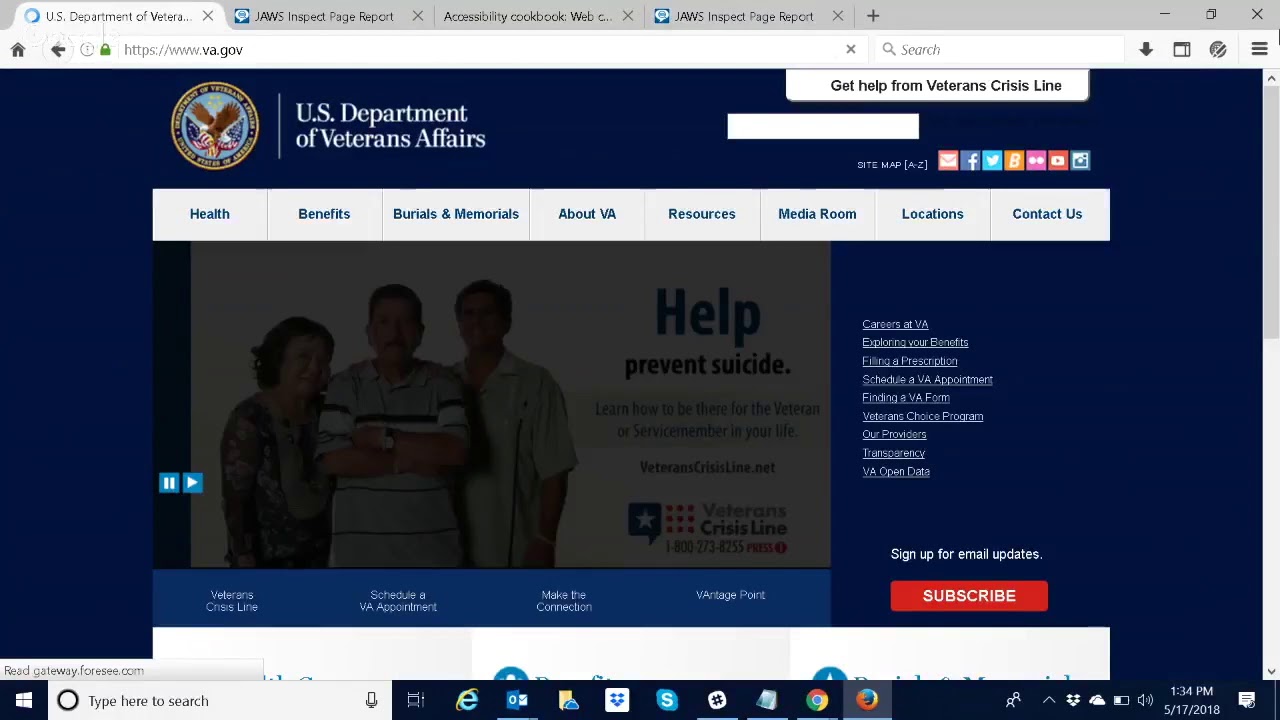The screenshot captures a web browser with four open tabs. The active tab displays the U.S. Department of Veterans Affairs website, located at www.va.gov. Prominently visible is the official government logo featuring an eagle flanked by American flags. In the upper right corner, there's a search bar, a tab labeled "Get Help from Veterans Crisis Line," a site map option, and various social media icons for platforms like Facebook and Twitter.

Below this section is a thick, white menu bar that is centered within the site's design but does not span the full width of the screen. This menu bar is segmented by gray dividers and features blue-text options including Health Benefits, Burials and Memorials, About VA, Resources, Media Room, Locations, and Contact Us.

Further down, the page features an image of three individuals: a man with his arms crossed standing in the center, a woman to his left, and another man to his right. Overlaid text urges to "Help Prevent Suicide," accompanied by a darkened background and a pause/play button suggesting video content. Beneath this, there are four text options that are too small to discern clearly.

To the right, a red "Subscribe" button invites users to "Sign Up for Email Updates," with additional menu text options nearby. The bottom of the screenshot shows the Windows 10 taskbar, complete with the search field, application icons, and system widgets in the bottom right corner.

Adjacent browser tabs include JAWS Inspect Page Report, Accessibility Cookbooks, and another JAWS Inspect Page Report, indicating an accessibility-focused browsing session.